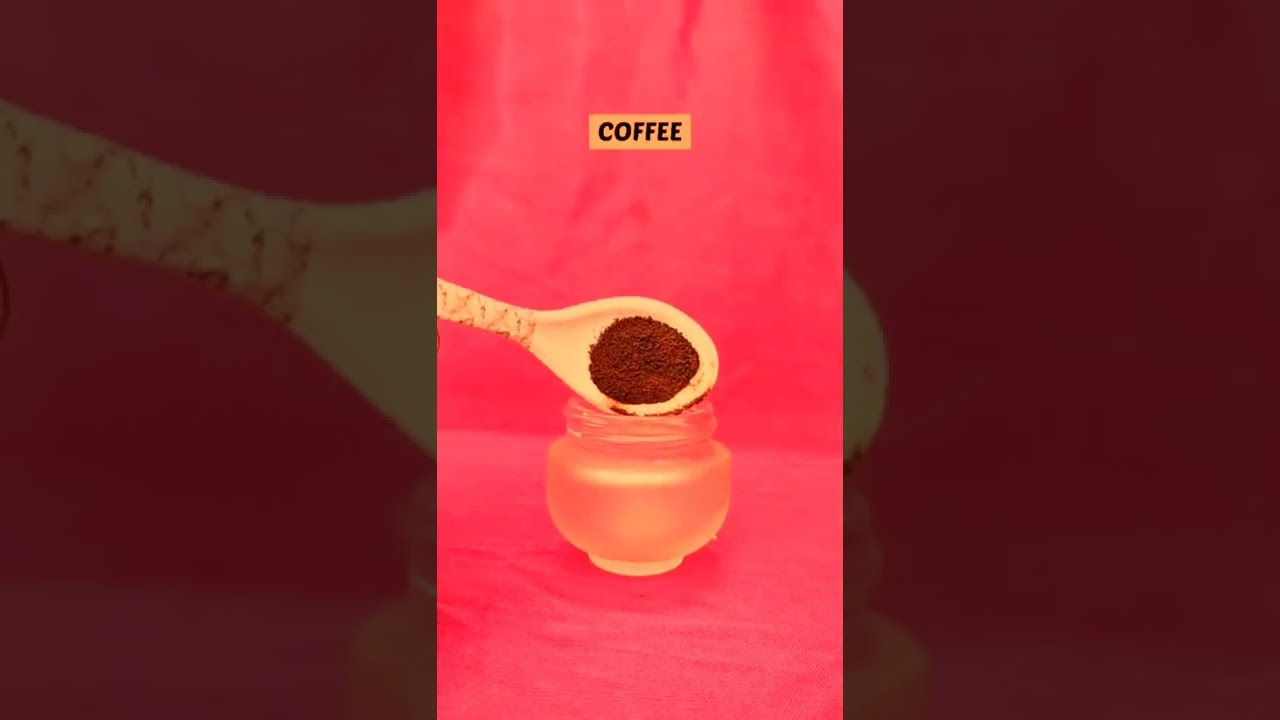The photograph, likely taken with a smartphone given its vertical cropping, captures a detailed scene centered around the theme of coffee. At the top of the image, the word "coffee" is displayed in small black text within a rectangular beige box, prominently positioned in the center. Below this, a wooden spoon, entering from the left side, holds brown coffee grounds and is poised above a small, transparent glass jar with a wide open neck, indicating grooves for a screw-on lid. The jar, appearing slightly frosted, rests on a vividly bright red surface, which also dominates the background, giving the impression of a red curtain. The spoon seems to hover or rest on the jar's edge, ready to pour its contents. The image is flanked by wide, shadowy borders on the left and right, created by enlarging and graying out elements of the central image, adding a dramatic framing effect. The overall composition, with its vibrant colors and focused subject matter, resembles an advertisement for coffee.